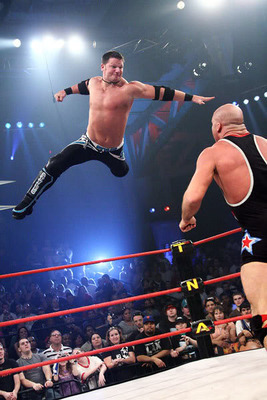In this vivid indoor photograph taken from inside a wrestling ring, a dynamic scene unfolds. The ring is partially visible in the lower right corner, featuring a white mat and three red ropes connected to a black turnbuckle pad with the yellow letters "TNA" vertically aligned. Dominating the foreground, a bald wrestler of Caucasian descent stands tensely in a black unitard adorned with a star on his left hip—the star edges in blue, transitioning to white, with a central red star. Mid-air above the ring, another Caucasian wrestler with short brown hair, shirtless, clad in long black pants with blue and white accents, black wrestling boots, elbow guards, and wristbands, appears to be executing a flying Superman punch. His fist is drawn back, ready to strike the wrestler below. The background reveals a crowd of spectators lit with a bluish hue under the stadium's tall ceiling, with a spotlight beaming down on the intense action in the ring.